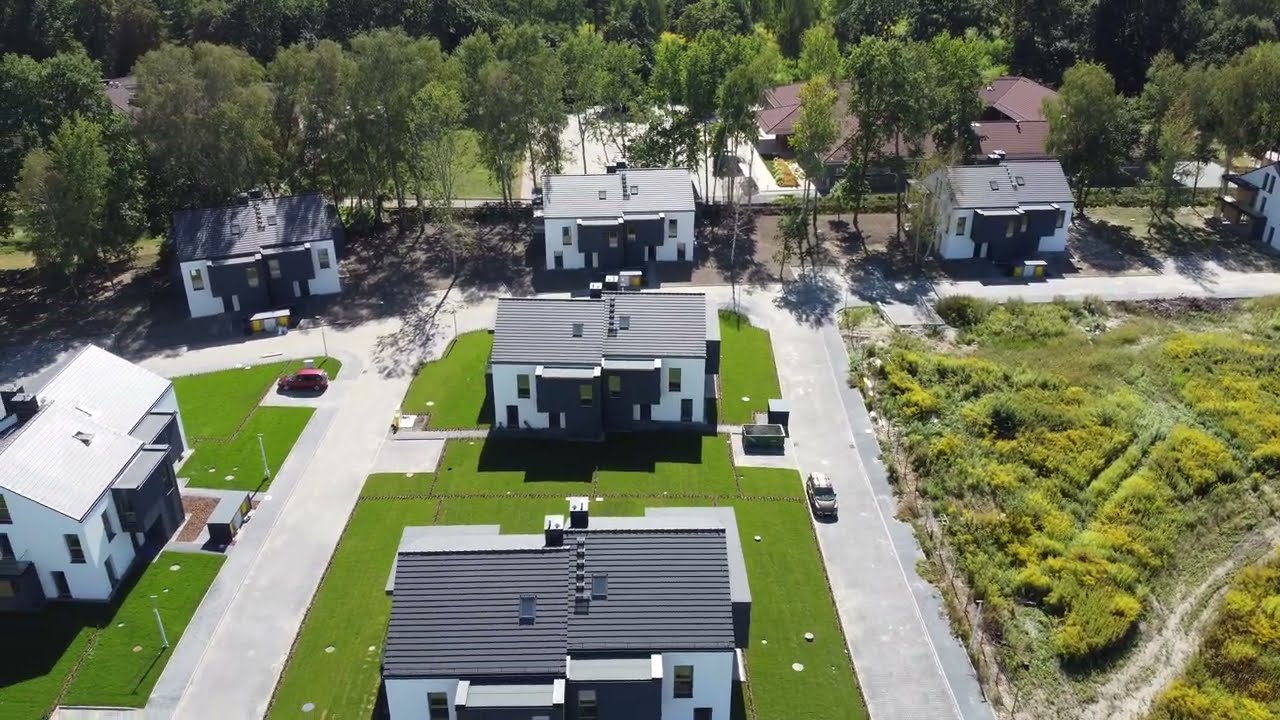This overhead view photograph captures a neatly arranged residential neighborhood featuring two-story houses with distinctive gray metal roofs and white and black exterior walls. Each house prominently displays multiple windows, with the upper floors featuring two windows per facade and the lower floors featuring four. The central house boasts two offset balconies, adding an element of architectural interest. Surrounding the homes is meticulously kept grass, bordered by a circular gray road that connects to another road running horizontally.

The foreground reveals a lush green field filled with various shades of vegetation and a noticeable beaten trail cutting through it. In the background, a towering line of thin-stemmed trees with thick foliage frames the scene, transitioning into a denser, darker forest at the far distance. Additional buildings with distinctive arched red roofs appear in the upper right corner, hinting at another neighborhood. On the street adjacent to the houses, a red car is parked in a small cut-out on the left side, and another vehicle is situated on the right.

Overall, the image provides a comprehensive view of the landscape, detailing the houses, greenery, and the layout of the roads, captured under a canopy of varying green hues.